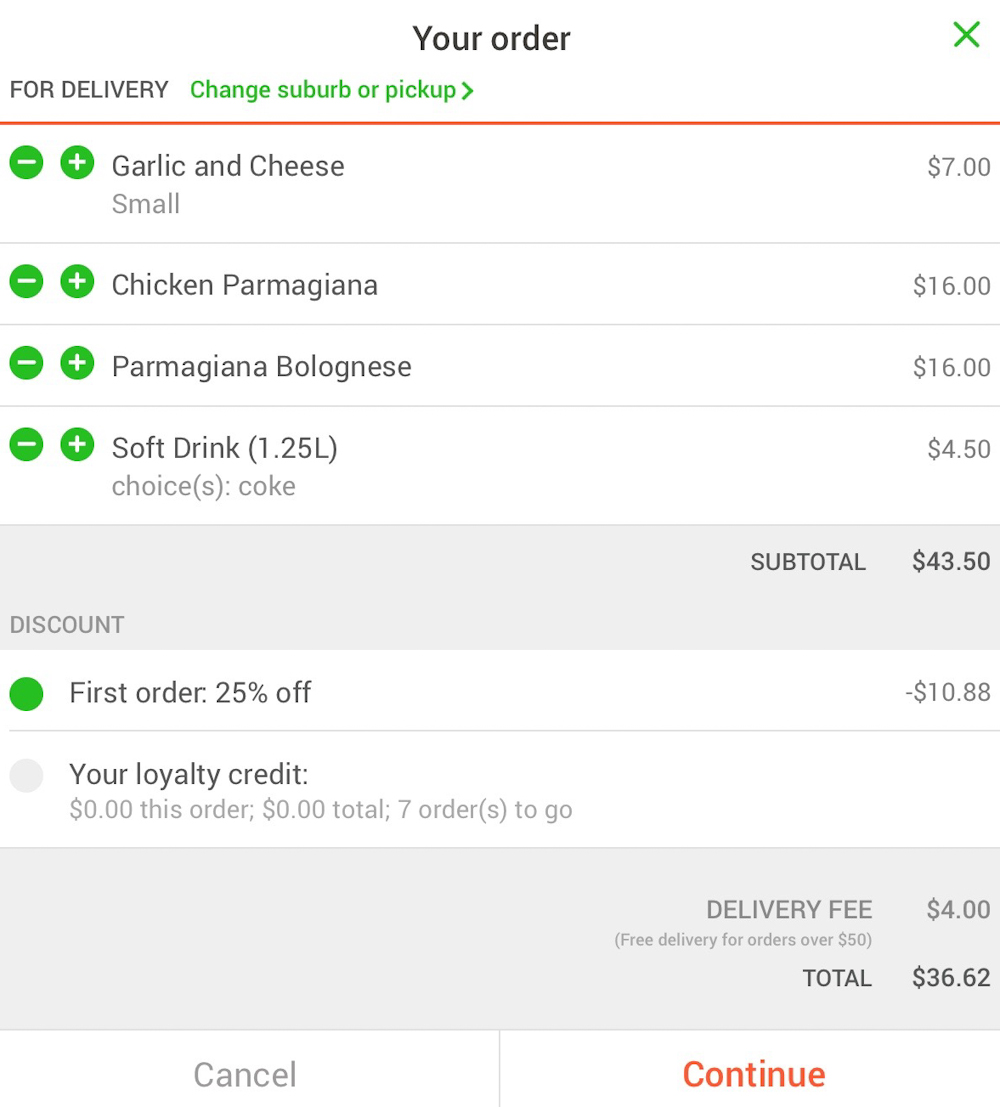The image is a screenshot of a food delivery order, likely from a service like DoorDash. The background is white, providing a clean and uncluttered look. At the top of the screenshot, there is a bold black header that reads "Your Order" with a green "X" icon to the right, likely for closing the order window.

The details of the order are listed below the header: 
- A small Garlic and Cheese item priced at $7. 
- A Chicken Parmesan priced at $16. 
- A Parmesan Bolognese also priced at $16. 
- A 1.25-liter soft drink, specified as Coke, priced at $4.50.

At the bottom of the list, there is a light gray box displaying the order summary. The subtotal is listed in bold black text as $43.50. Below, there is a section for discounts, showing that a 25% off discount on the first order has been applied. This discount is indicated by a green bubble and the deduction of $10.88.

Further down, the delivery fee is noted. It states that delivery is free for orders over $50; otherwise, there is a $4 delivery fee. For this order, which totals $36.62 after discounts, the delivery fee applies.

At the very bottom of the screen, there are two buttons: "Cancel" on the left and "Continue" on the right, with the "Continue" button highlighted in orange.